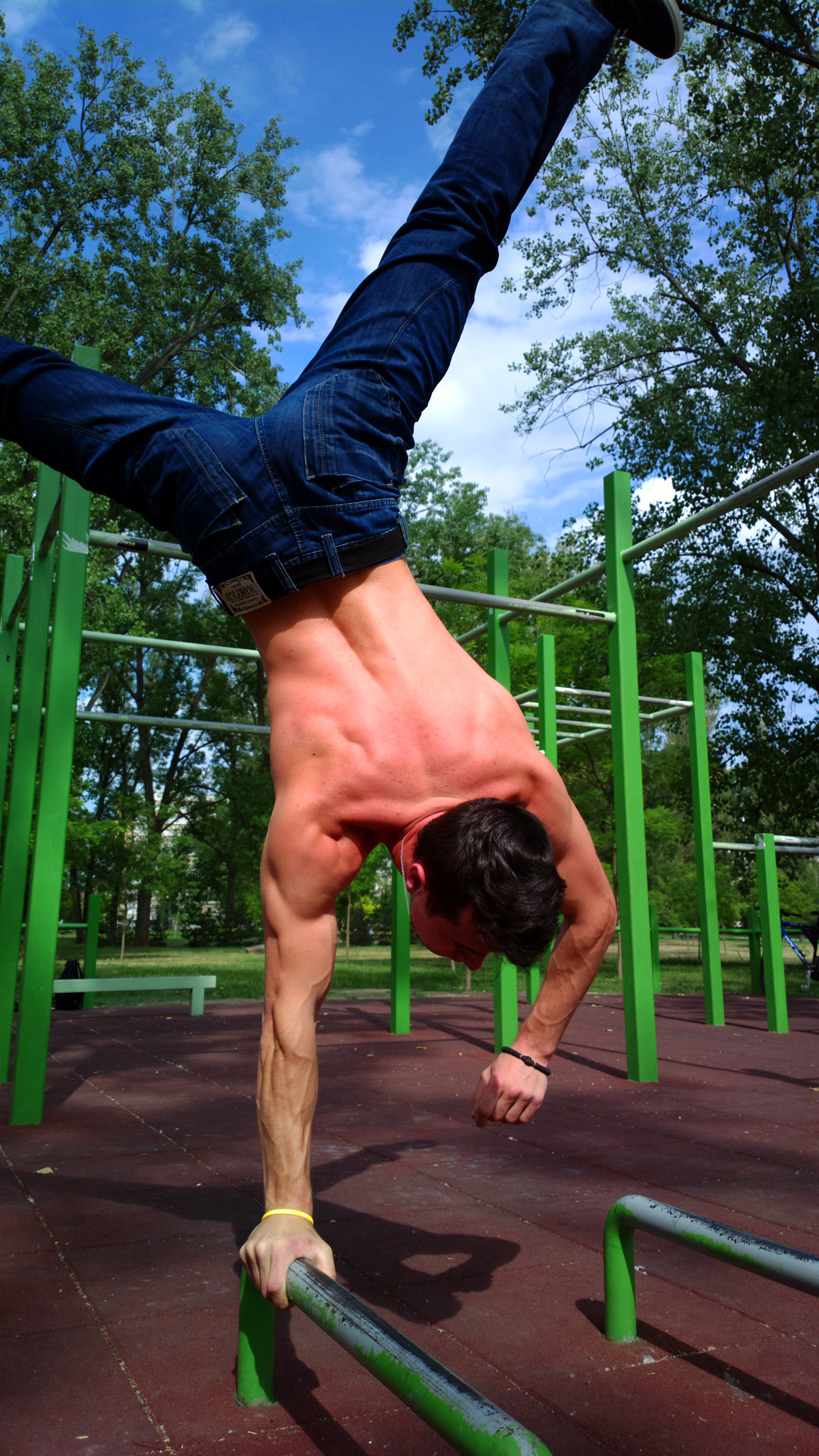This is a photograph of a man performing an impressive one-handed handstand on a small green rail in a playground or exercise area. The man, shirtless and wearing blue jeans, displays notable muscular strength as he balances on his right hand with his legs spread apart in the air. He sports a yellow bracelet on his right wrist and a black bracelet on his left. The playground surroundings include various green metal apparatus like monkey bars and balance beams, some of which show signs of wear. The rails emerge from a red, spongy ground surface, typical of safety flooring in such areas. Behind the playground, a clear blue sky and an array of trees enhance the scenic, tranquil atmosphere. Despite the typically child-friendly equipment, there are no children present, just the man showcasing his gymnastics-like skills.